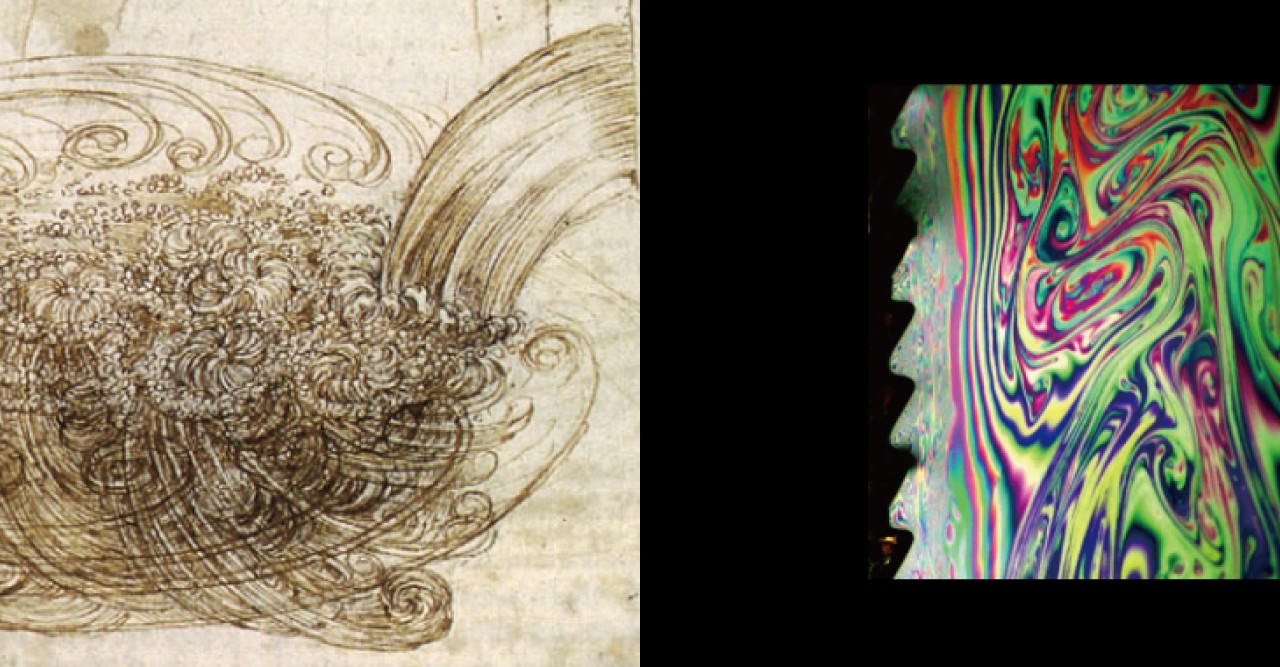The image is divided into two panels. The left panel features an old-fashioned, off-white, cream-colored background with intricate sketches rendered in blacks and deep browns. The artwork represents flowing lines that abstractly resemble water or wind, interspersed with circular patterns that converge into a central vortex-like structure. The right panel contrasts sharply with a solid black background, showcasing an abstract, colorful object with vibrant hues of green, red, purple, and blue. This multicolored object, resembling a kaleidoscope or the iridescent sheen of a bubble, appears almost as a swirl of unmixed paints or a computer-generated image. The juxtaposition of the two diverse artistic styles—the delicate, ancient-feeling sketch on the left and the bold, modern abstraction on the right—creates a compelling visual narrative.